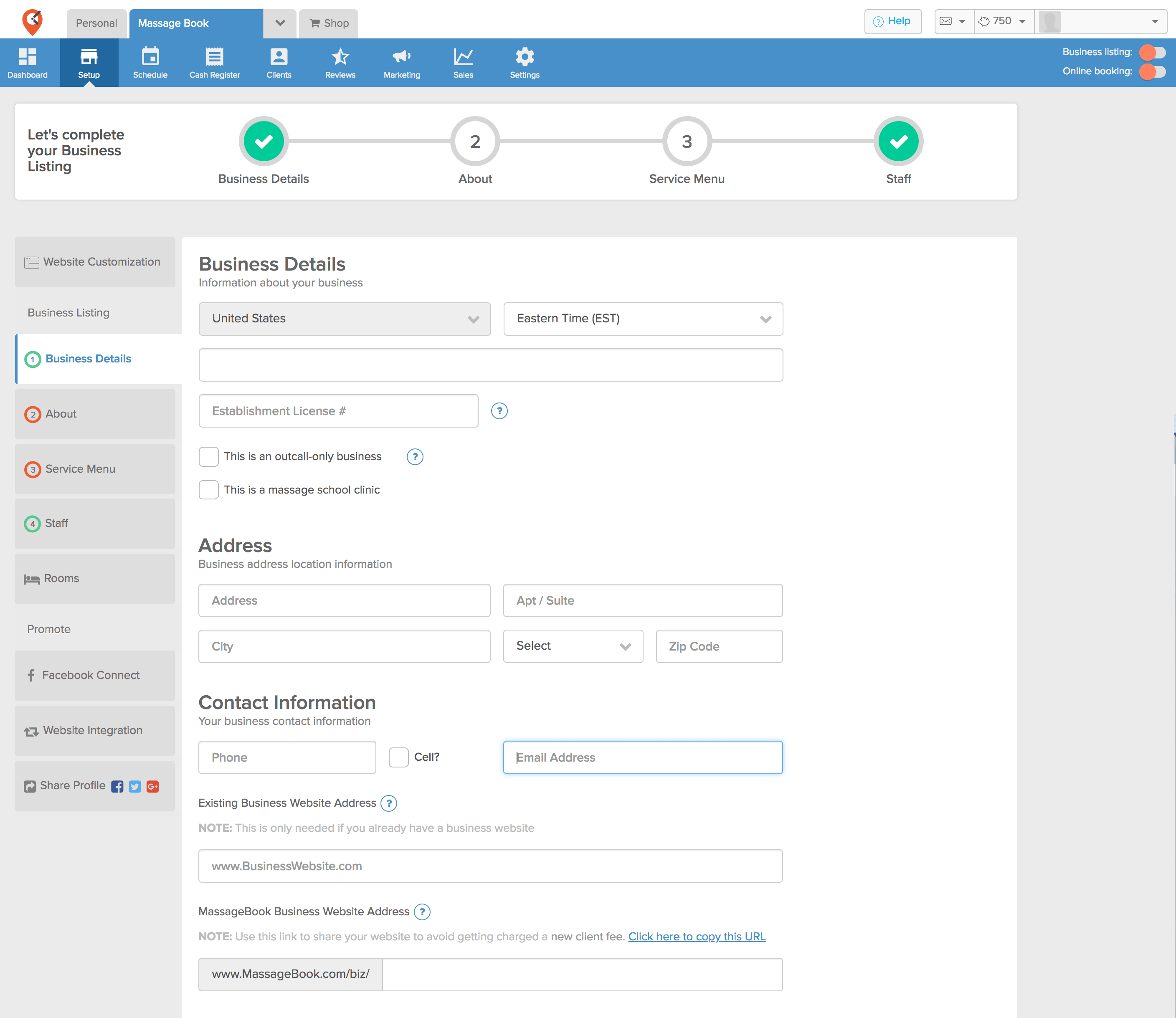A detailed photograph of a business listing web page showcases various sections and elements aimed at helping users complete their business profile. In the top left corner, tabs labeled "Personal," "Message Book," and "Shop" are visible, indicating different functionalities of the platform. Beneath these tabs, a blue-bordered navigation menu features options such as "Dashboard," "Setup," "Schedule," "Cash Register," "Claims," "Reviews," "Marketing," "Sales," and "Settings."

Centrally, the page prompts users to "Let's Complete Your Business Listing," outlining a multi-step process. Step 1 is titled "Business Details," Step 2 is labeled "About" with a circle indicating its sequence, Step 3 is "Service Menu," and the final step, marked with a green circle and a white check mark, is "Staff."

On the far left, a vertical column lists additional sections: "Website Customization," "Business Listing," "Business Details," "About," "Service Menu," "Staff," "Rooms," "Promote," "Facebook Connect," "Website Integration," and "Share Profile."

To the right, the section focuses on "Business Details" encompassing fields for "Information About Your Business." It specifies the geographical context with "United States, Eastern Time." There's a field for "Establishment License Number" accompanied by a circle with a question mark icon for additional information. Options for "This is an out-call only business" and "This is a massage school clinic" are present with unchecked boxes for user selection.

Further down, the form requests "Address" details with labeled rectangular boxes for "Business Address Location Information." The boxes are marked for "Address," "Apartment/Suite," "City," "State" (selectable via a downward arrow), and "Zip Code." Beneath this, the section titled "Contact Information" seeks "Your Business Contact Information" with designated boxes for "Phone" and "Email Address."

This thorough and user-friendly layout guides business owners through the steps required to furnish their listing with essential and comprehensive details.